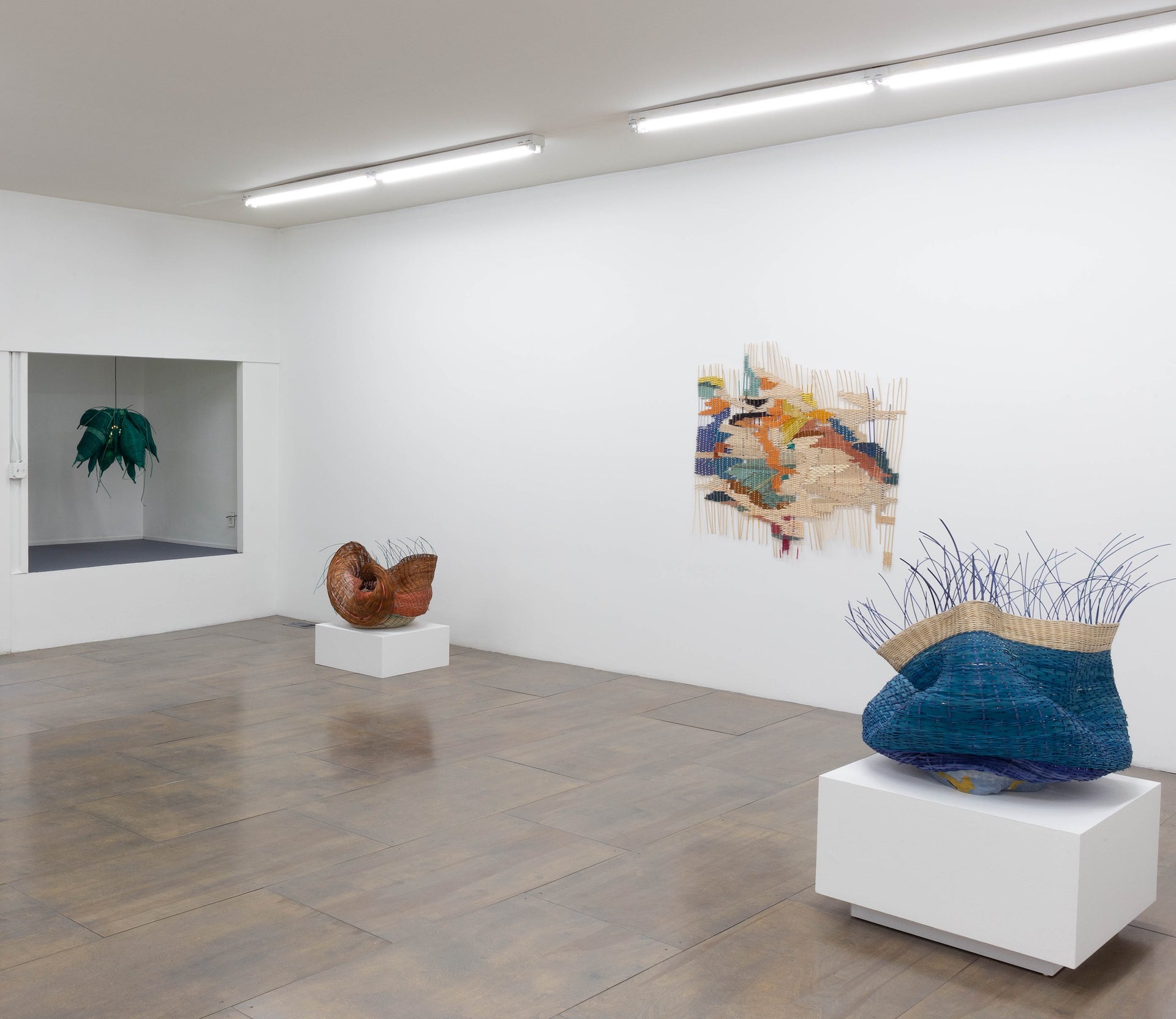The image depicts the interior of an art museum, characterized by a minimalistic design with predominant white walls and ceiling. The space is well-lit by two long, thin fluorescent lights mounted at the top. Centered on the back wall is a vibrant, multicolored abstract painting displayed on a white wall. Adjacent to the painting on the left wall is a recessed display niche containing an art object. Dominating the left side of the image is a very full and vivid green hanging plant, contributing a touch of nature to the scene.

On the left corner of the image, a white cube pedestal supports a brownish-orange woven object, which appears to be a basket or a similar artifact. Matching this setup, another white cube pedestal is positioned at the bottom right corner, adorned with a navy blue basket that features a beige fringe detail.

The space derives warmth from a richly colored, brown wooden floor that harmonizes with the brown elements in the artwork and artifacts, subtly breaking the dominance of white. The diverse array of colors—green, brown, blue, yellow, orange, red, and light blue—adds vibrancy to this meticulously curated museum exhibit, giving depth and interest to the setting.